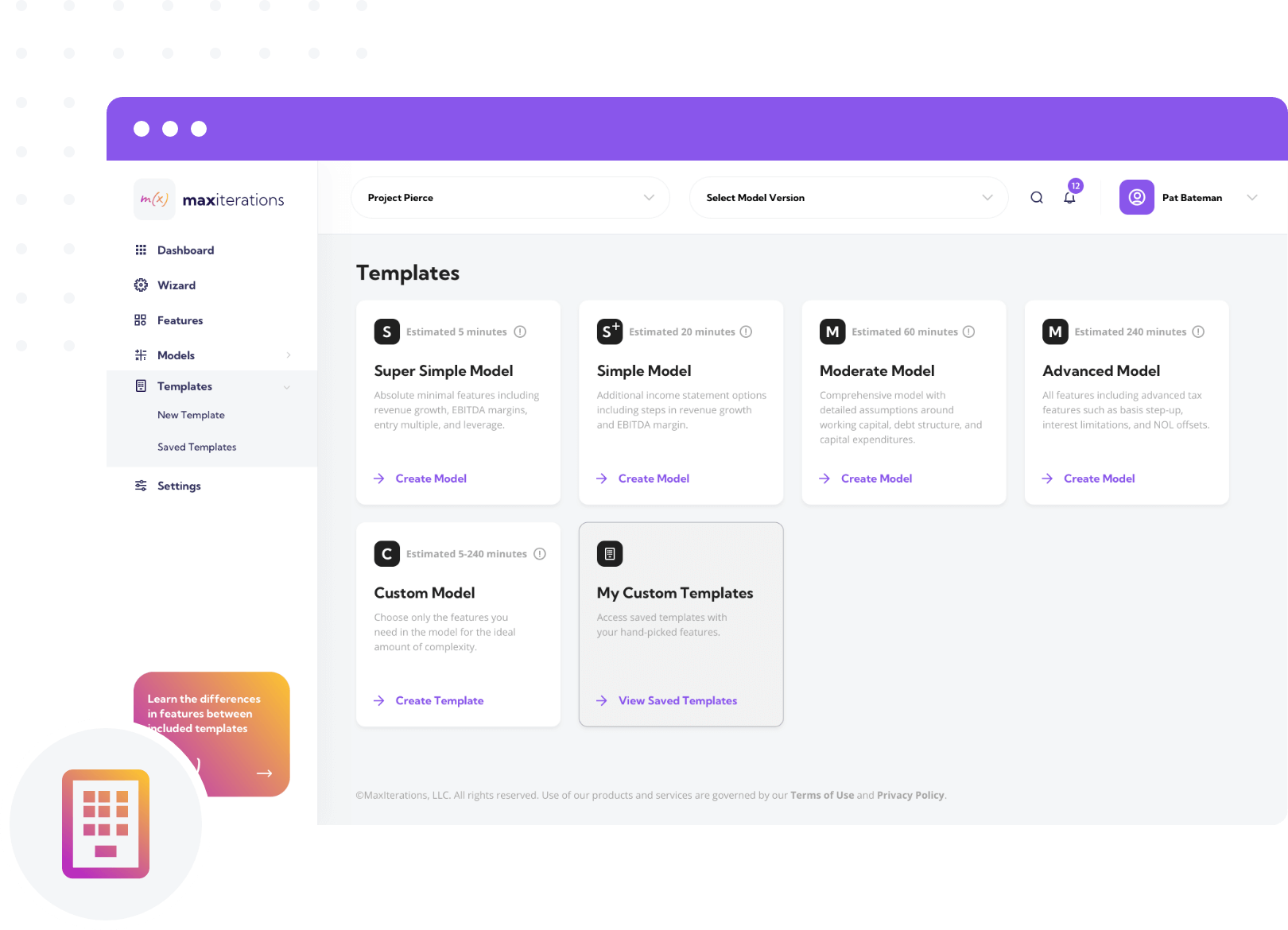This is a screenshot from an unknown interface displaying a dark purple banner at the top, which features three horizontal circles on the left side. Below the banner, a vertical drop-down menu on the left lists options: Dashboard, Wizard, Features, Models, Templates (selected), New Template, Save Templates, and Settings. 

On the right, the header includes "Project Pierce," a drop-down for "Select Model Version," a notification icon with 12 alerts, a search icon, and the user name "Pat Bateman."

The main section is divided into different modeling options:

- **Templates:**
  - **Super Simple Model:** Estimated 5 minutes to create; includes minimal features like revenue growth, EBITDA margins, entry multiple, and leverage. Option to "Create Model."
  - **Simple Model Plus:** Estimated 20 minutes to create; includes additional income statement options and revenue growth alongside EBITDA margins. Option to "Create Model."
  - **Moderate Model:** Estimated 60 minutes to create; a comprehensive model with detailed assumptions around working capital, debt structure, and capital expenditures. Option to "Create Model."
  - **Advanced Model:** Estimated 240 minutes to create; covers all features, including advanced tax aspects like basis, step-up, interest limitations, and NOL offsets. Option to "Create Model."

- **My Custom Templates:** Allows access to saved templates with handpicked features. Option to "View Saved Templates."

At the bottom of the screen, it reads: "Copyright maxiterations LLC, all rights reserved. Use of our products and services are governed by our terms of use and privacy policy."